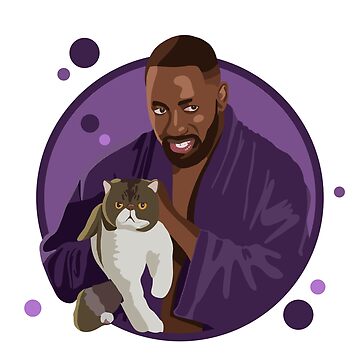The image is a detailed, illustrated logo featuring an African American man holding a Siamese cat. The logo is circular, filled with violet, and edged with dark purple. Surrounding the circle are five varying purple dots, ranging from light to dark shades. Inside the circle, the man, dressed in a purple bathrobe, cradles the cat with its white body and brown head. The cat has striking yellow eyes. The man, depicted with dark, close-cropped hair, is looking off to his left (our right) and is not smiling but showing his teeth. The illustration, reminiscent of an old-style Adobe Illustrator approach, employs layered techniques without any text in the image, featuring predominant colors of purple, white, brown, black, and gray. The overall style is a digital drawing or computer-assisted illustration, portraying the man in a calm, serene moment with his pet.